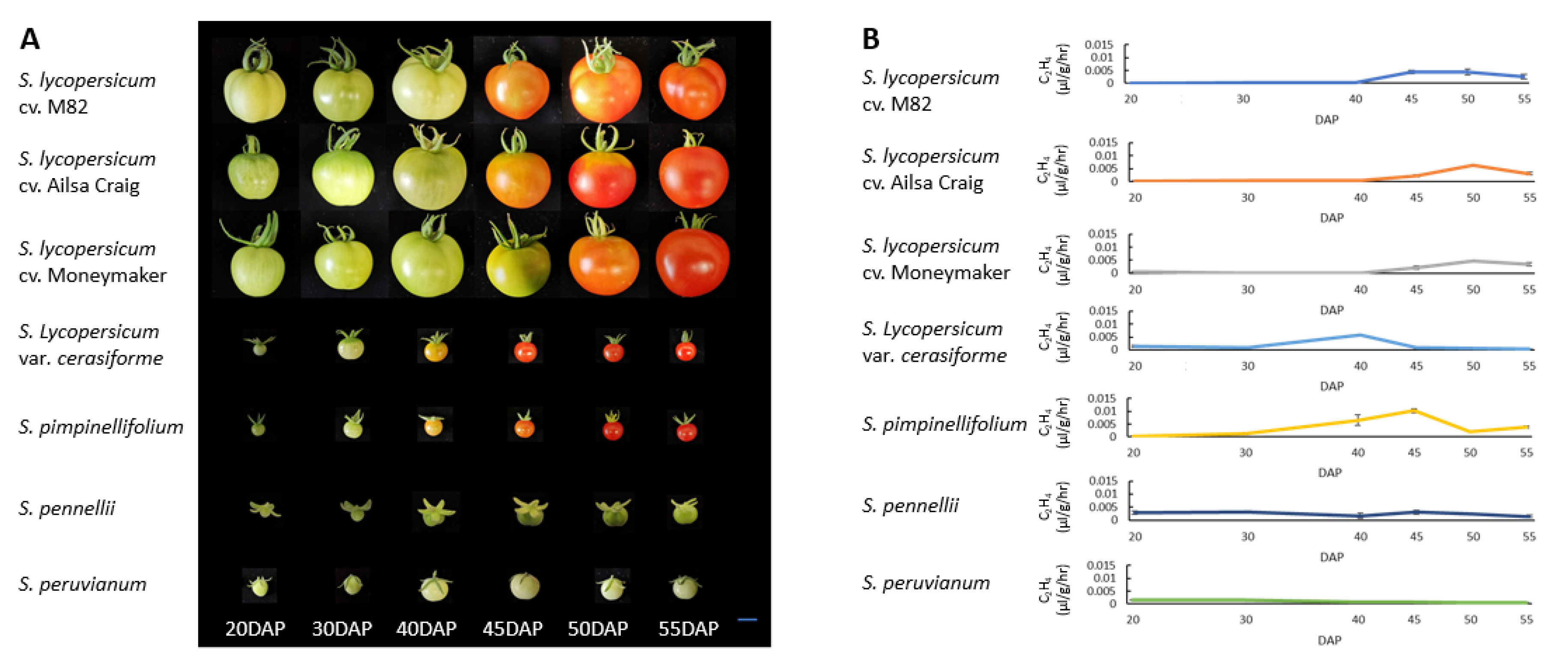The image is a rectangular illustration comprised of two sections, labeled A and B, which depict different aspects of the growth cycles of tomato plants. The left section, labeled A, features a visual progression of tomato ripeness through various stages—from green to orange to red—set against a black background. Each row of images in this section is accompanied by lines of black text listing several Latin names: A, S. lycopersicum CVM82, S. lycopersicum CV Elsa Craig, S. lycopersicum CV Moneymaker, S. lycopersicum VAR Sarasviform, S. pimpinilifolium, S. pinelli, S. peruvianum. The right section, labeled B, contains detailed graphs corresponding to each row of text from section A, providing a statistical perspective on the growth. Together, the charts offer a comprehensive visual and quantitative analysis of tomato plant growth cycles.